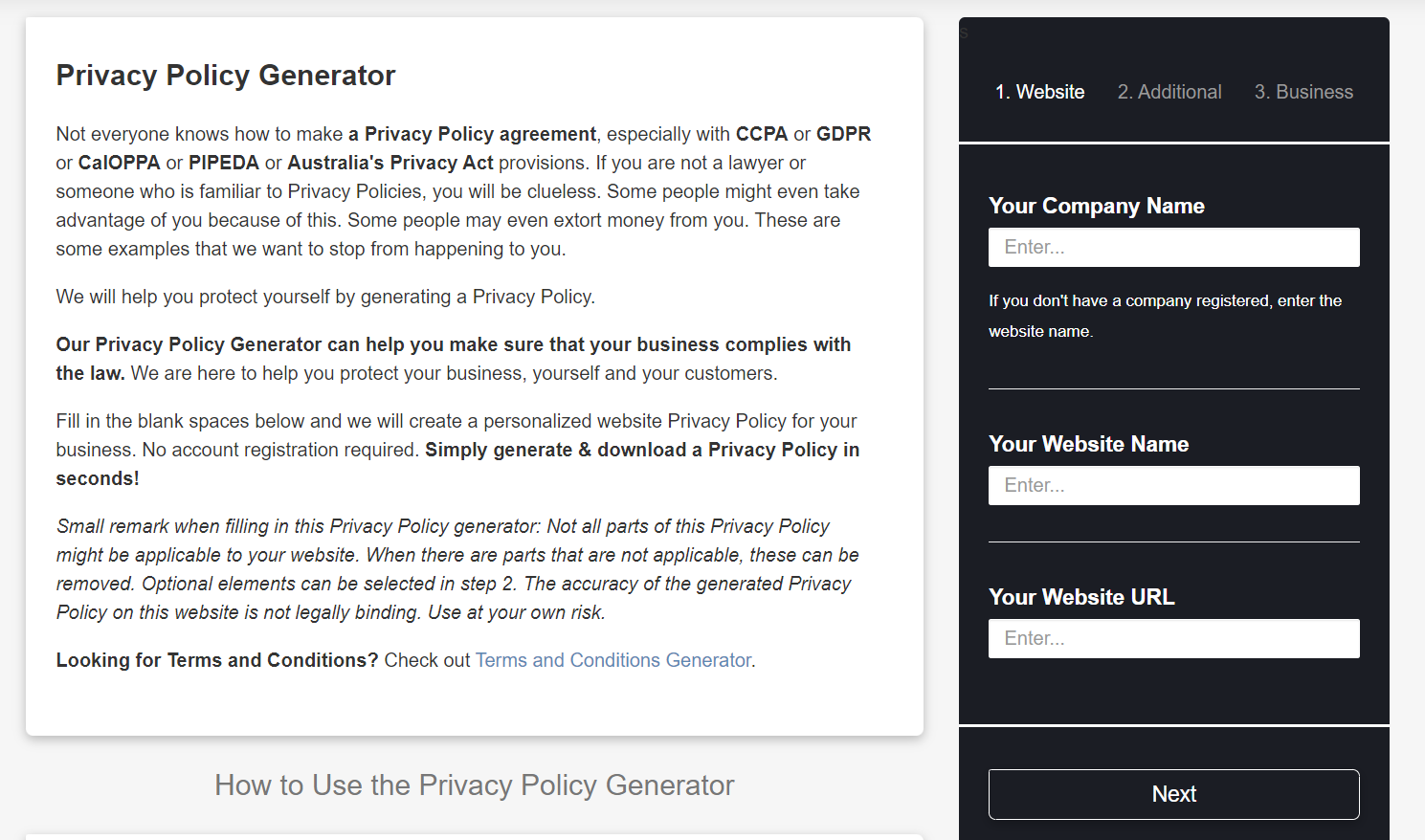The image depicts a user interface for a "Privacy Policy Generator" website. The interface is divided into two sections. On the left, an explanation highlights the complexities of creating a comprehensive privacy policy, especially considering regulations such as CCPA, GDPR, CALOPPA, PIPEDA, and Australia's Privacy Act. It emphasizes the risks of not being knowledgeable about privacy policies, including potential exploitation and financial extortion. The text assures users that the generator will help them create a compliant privacy policy to protect their business, themselves, and their customers. 

On the right, there are three selectable options: "Website," "Additional," and "Business." The currently selected option is "Website." Beneath it, the user is prompted to enter their "Company Name" with a field provided for this input. If the user does not have a registered company, they are instructed to enter their website name instead. Following this, additional fields are available for entering the "Website Name" and "Website URL." At the bottom of this section, there's a "Next" button for proceeding to the next step.

The explanatory text also includes a disclaimer, stating that the generated privacy policy may not be legally binding and should be used at the user's own risk. Users are cautioned that not all elements of the generated policy may apply to their website, and they have the option to remove inapplicable sections or choose optional elements in Step 2. The process does not require account registration and allows users to generate and download their privacy policy quickly.